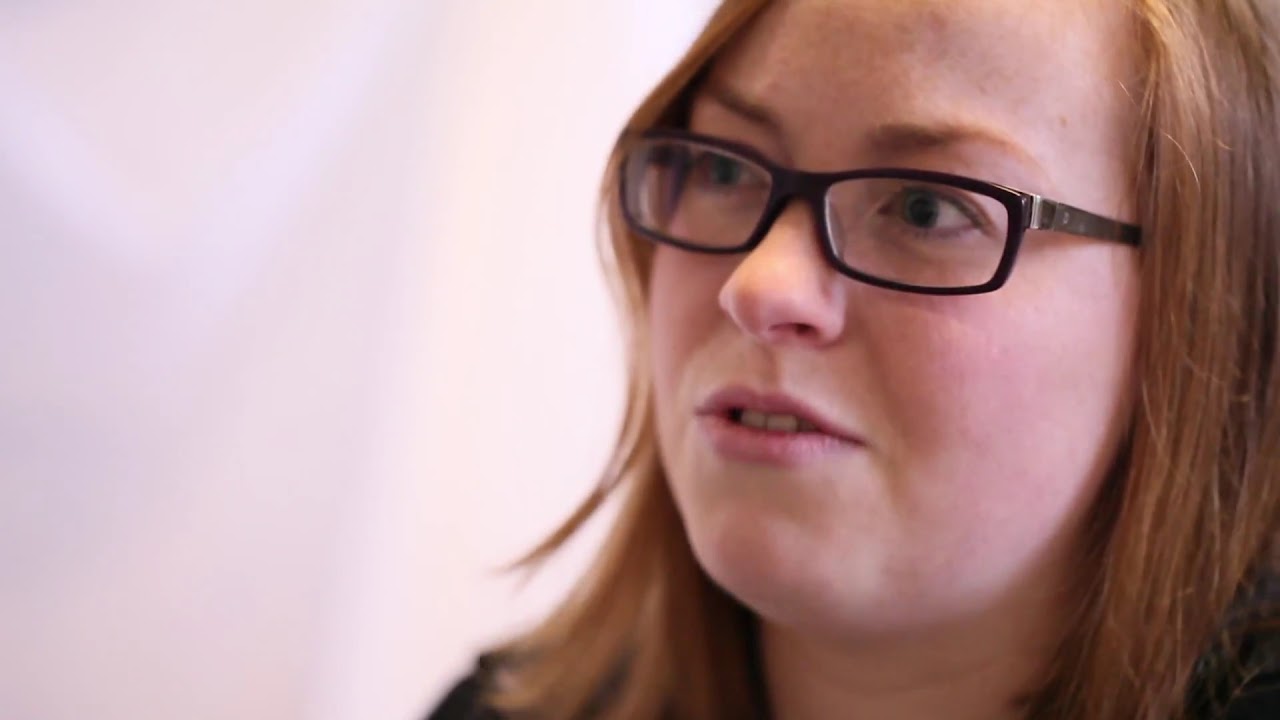This color photograph captures a close-up of a woman's face with a predominantly white background. She has red, shoulder-length hair that is straight and slightly swooped over her black-rimmed glasses. Her eyes, which are blue, are looking towards the left. The woman has reddish eyebrows, a prominent nose, and visible freckles on her forehead, accentuated by rosacea-dotted skin. She is wearing a black top, though only part of it is visible. Her lips are chapped and naturally pink, with her mouth slightly open, showing her two front teeth. The image composition places the woman predominantly on the right half, creating significant negative space on the left.